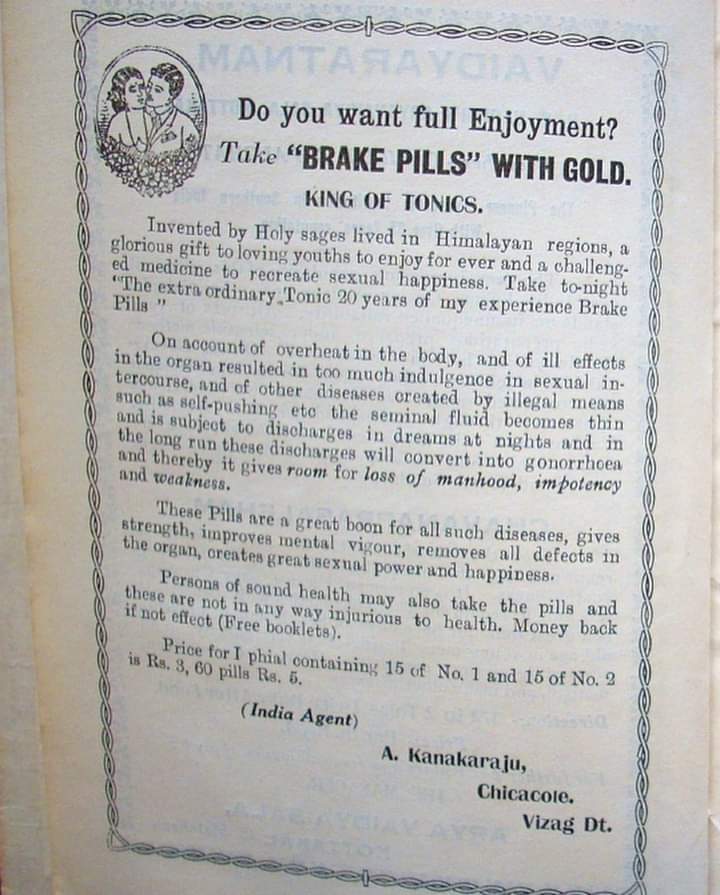The image is an old advertisement, possibly from a newspaper or magazine, featuring an illustration in the top corner of a man kissing a woman on the cheek against a backdrop of foliage. The advertisement prominently displays the text: "Do you want full enjoyment? Take 'Break Pills' with Gold, King of Tonics." It claims these pills were "invented by holy sages who lived in the Himalayan regions," and describes them as "a glorious gift for loving youths to enjoy forever and a challenged medicine to recreate sexual happiness." A paragraph elaborates, stating: "On account of overheat in the body and of ill effects in the organ resulted from too much indulgence in sexual intercourse and other diseases created by illegal means such as self-pushing, the seminal fluid becomes thin and is subject to discharges in dreams at night. In the long run, these discharges will convert into gonorrhea, thereby giving room for loss of manhood, impotency, and weakness." The advertisement promotes the pills as an extraordinary tonic, touting 20 years of experience, and indicates it's marketed by an agent named A. Kanakaraju from Chikakote, Vizagditi, India. Despite its grandiose claims, the pills are likely ineffective according to modern scientific standards.